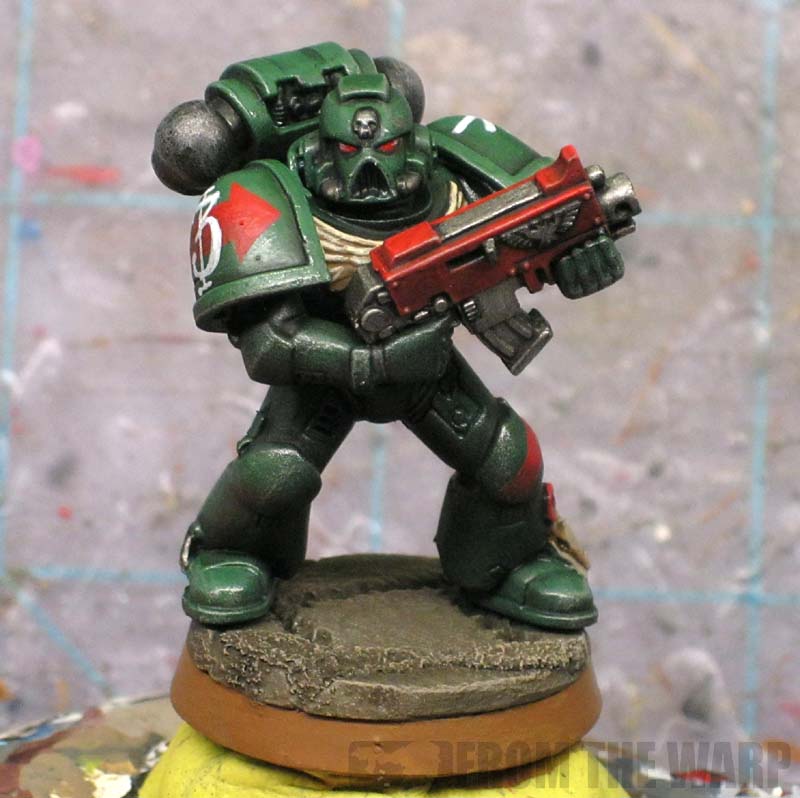The image captures a Warhammer 40k miniature figurine, accentuating the detailed craftsmanship of the character. The backdrop appears to be a gray, cement-like wall, adorned with an array of speckled white dots, light blue lines, and splashes of red, pink, and blue paint, providing a colorful contrast. The figure stands on a rugged, circular stone base, suggesting a staged battlefield setting. In the bottom-left of the background, hues of tan, reddish colors, and white are visible, along with a yellow section directly beneath the toy.

Dominating the scene, the miniature is an imposing robotic soldier clad in green and gray armor, evoking the menacing atmosphere of the Warhammer 40k universe. The armor is intricately detailed, featuring a silver skull on the helmet, piercing red eyes, and a black-barred mouthpiece. A red arrow and a white bee are marked on its right shoulder, further embellishing its warlike appearance. Its chest is protected by a white plate, with a black torso piece beneath. The miniature wields a red and silver gun in an aggressive stance, right finger on the trigger and left hand supporting the barrel. Additionally, the bottom-right corner of the image includes a smaller robot holding a gun, with the caption "FROM THE WARP" in gray text, adding context to the figurine's origin within the Warhammer 40k lore.